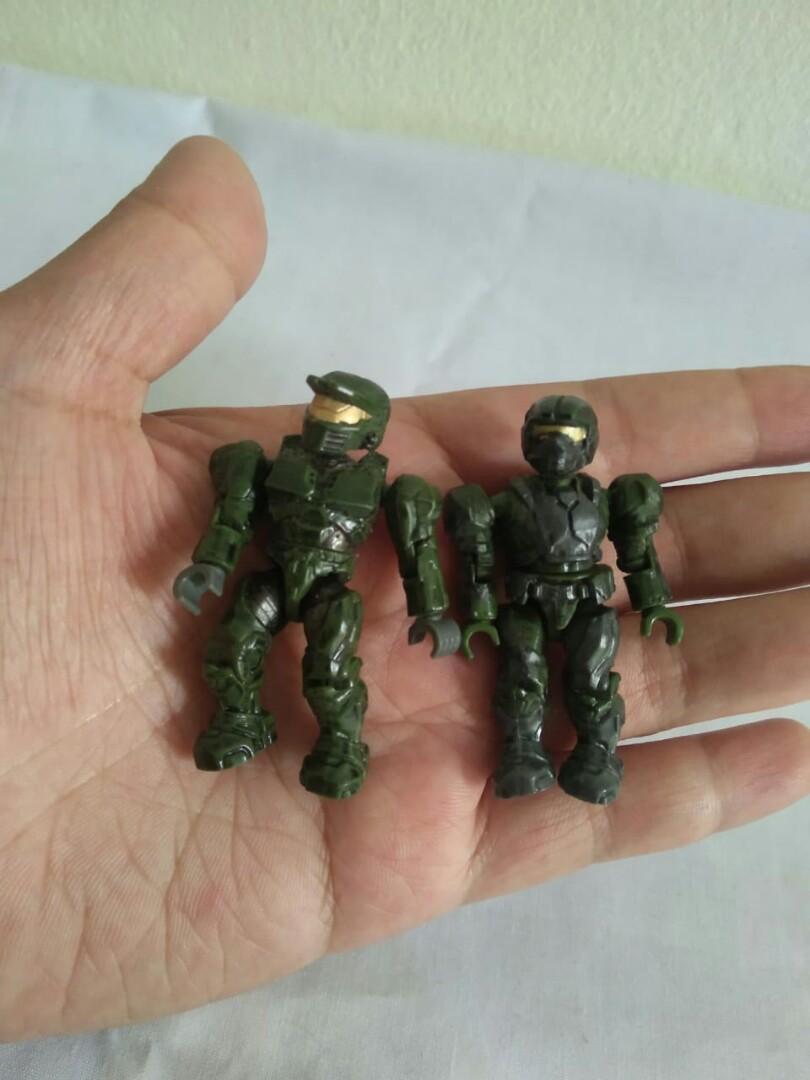The detailed image captures a close-up of a Caucasian person's left hand, opened palm-up, holding two small military action figures. The backdrop consists of a crumpled white piece of paper with a cream-colored wall visible at the top of the frame. The hand, detailed with visible lines and creases, showcases the figures positioned side-by-side. These figures, resembling characters from the Microsoft Halo series, are dressed in olive drab green armor with matching helmets. The helmets feature a shiny gold visor covering where their eyes would be. Both figures have jointed, cupped hands typical of Lego-style components, suggesting they may belong to a specific set. They are approximately the size of three of the person's fingers, with one figure appearing slightly larger due to a differing helmet shape.